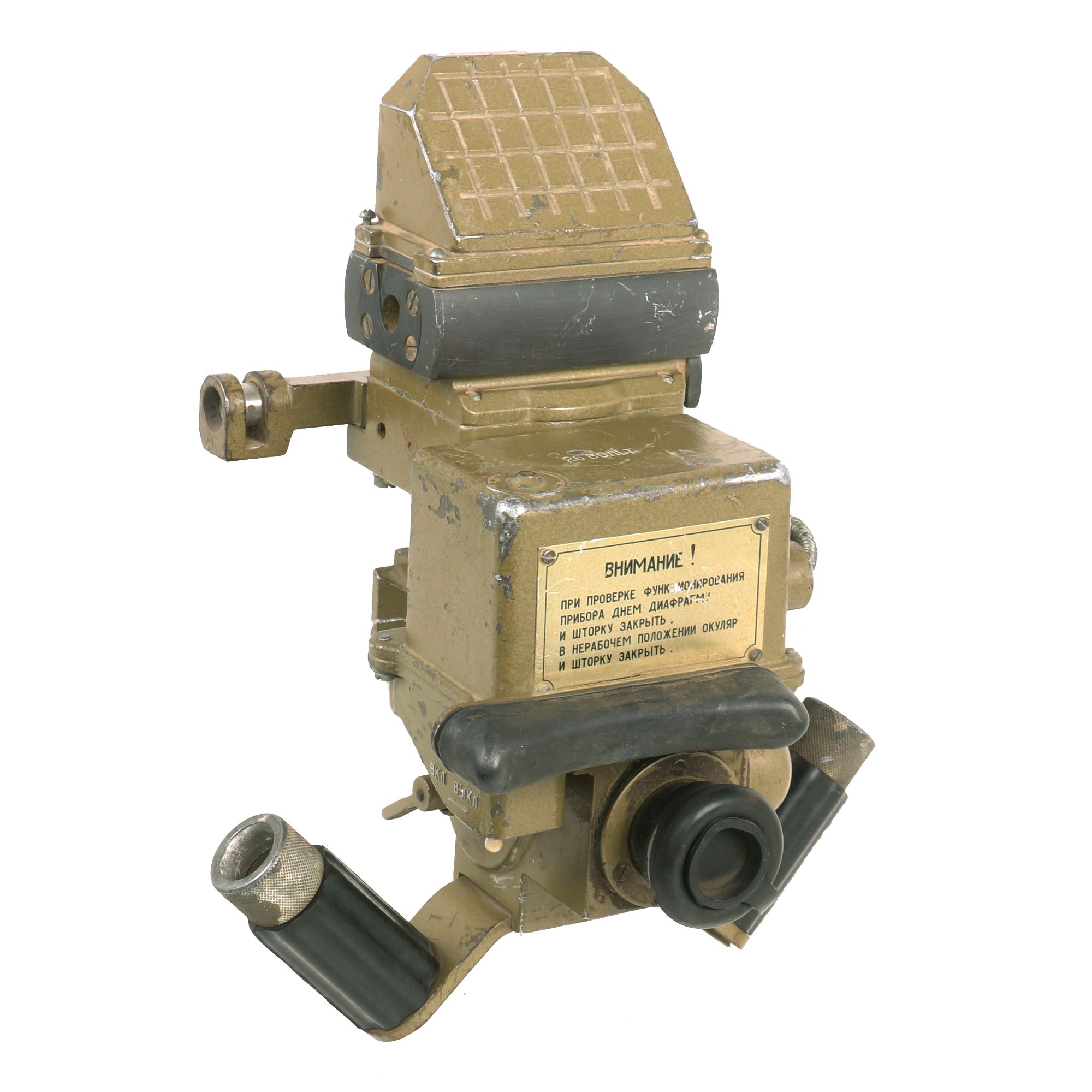The image is a full-color photograph of an aged and somewhat worn piece of metallic machinery, set against a plain white background. The device, predominantly painted in an army green hue with noticeable areas of chipped paint exposing the silver metal underneath, features various notable elements. At the top, it has a slightly sloped, square section with a lighter green grid pattern. Centrally located on the device is a cube-shaped box or plaque made of light copper metal, secured by screws at the corners. This plaque, bearing black text in a foreign language, serves as a focal point and includes an exclamation point followed by a list. The bottom section houses a black-edged lens, flanked on either side by black tubes each topped with a silver ring. Additional black rubber pieces, a knob, a handle, and attachment points that might be used for connecting hoses are also present, contributing to the machinery's intricate design.